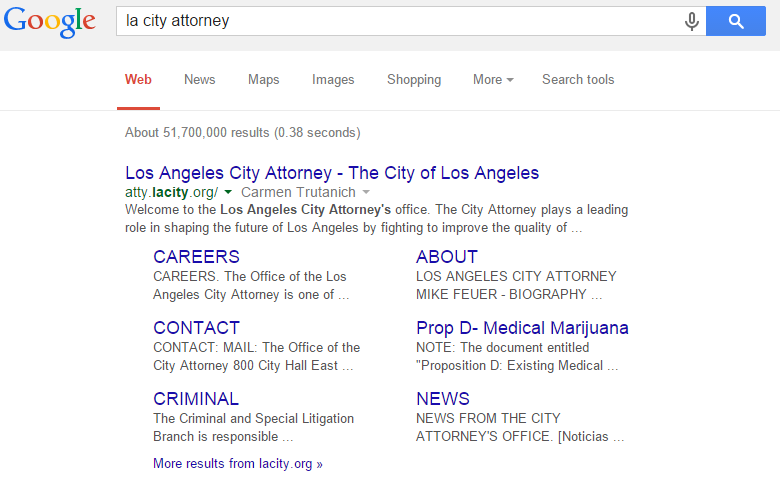Screenshot of a Google Search for "LA City Attorney":

In this screenshot, the Google homepage is prominently displayed with the familiar multi-colored Google logo positioned in the top left corner. The search query "LA City Attorney" is typed into the search bar centrally located at the top of the page. The search bar is flanked by a blue magnifying glass icon on the far right and a small microphone icon just to the left of it.

Below the search bar, the navigation tabs are visible, including options for "Web", "News", "Maps", "Images", "Shopping", and more—the "Web" tab is selected and highlighted in red. The search results indicate that there are approximately 51,700,000 results, retrieved in a rapid 0.38 seconds.

The first search result listed is from the official Los Angeles City Attorney's Office website, atty.lacity.org. The snippet from this result reads: "Welcome to the Los Angeles City Attorney's Office. The City Attorney plays a leading role in shaping the future of Los Angeles by fighting to improve the quality of...", before cutting off. Additional options below this result provide links to sections such as Careers, About, Contact, Prop D (referring to Proposition D related to medical marijuana), Criminal, News, and more results from LACity.org.

The screenshot captures an insightful moment where an individual has searched for information about the LA City Attorney and successfully found the relevant official page immediately. The mention of Proposition D implies a reference to legislation from the past, providing a slight context to the time frame of the search results.

Overall, this detailed snapshot showcases a user efficiently utilizing Google's search capabilities to obtain information about a key public office in Los Angeles.